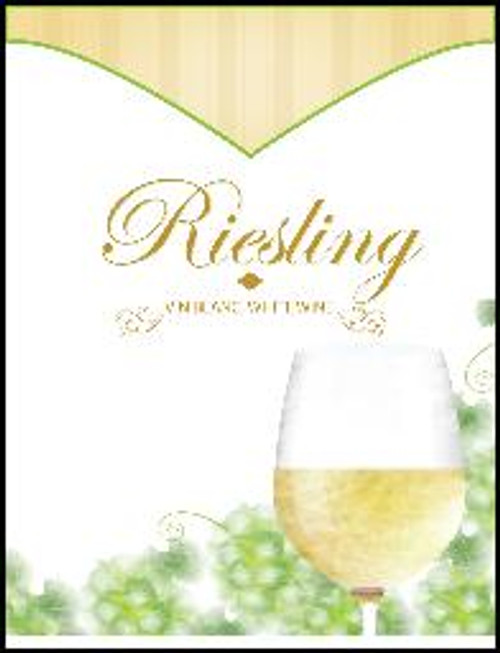The image, although of very poor quality and heavily compressed, appears to be a wine advertisement poster featuring a stemmed glass of Riesling wine. The top of the image includes a V-shaped banner outlined in lime green with golden and beige stripes. Beneath this, against a white background, the word "Riesling" is prominently displayed in a cursive gold font. Below this text, there is more illegible writing due to the image's low resolution. Towards the bottom right of the image, partially obscured, is a photograph of a wine glass filled halfway with a golden-hued white wine, showing only the upper part of the glass and a bit of the stem. The background behind the wine glass depicts blurry green plants or possibly a vignette of green grapes and leaves, suggesting a vineyard setting.